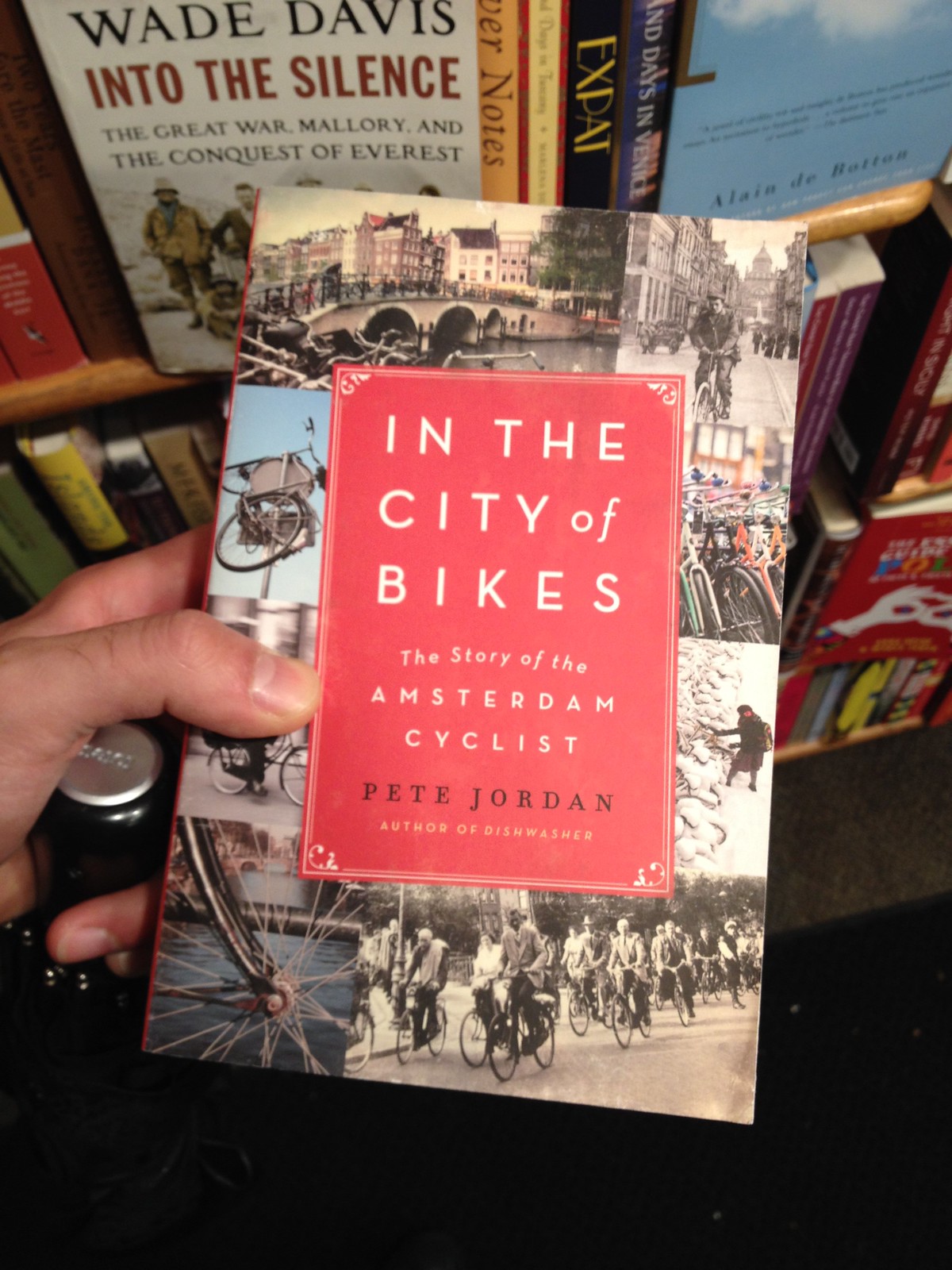In the foreground of the image, a hand is partially visible, with the thumb and second finger prominently grasping a book. The book, centered in the frame, is titled "In the City of Bikes: The Story of the Amsterdam Cyclist" by Pete Jordan. Its cover features a red background with the title in white text, and Pete Jordan’s name in black font. The subtitle "author of Dishwasher" is in smaller yellow font. Surrounding the title are images of people riding bicycles through various locations in Amsterdam, depicted in black and white. The perimeter of the cover is adorned with illustrations of bike spokes. Behind the hand holding the book, the scene expands to include shelves filled with books, suggesting the setting is a bookstore or library. Prominently displayed among the background books is Wade Davis’s "Into the Silence: The Great War, Mallory, and the Conquest of Everest," distinguishable amidst the rows of books, though other titles remain unreadable. The floor beneath the scene is black, contributing to the overall composition and ambiance of the scene.